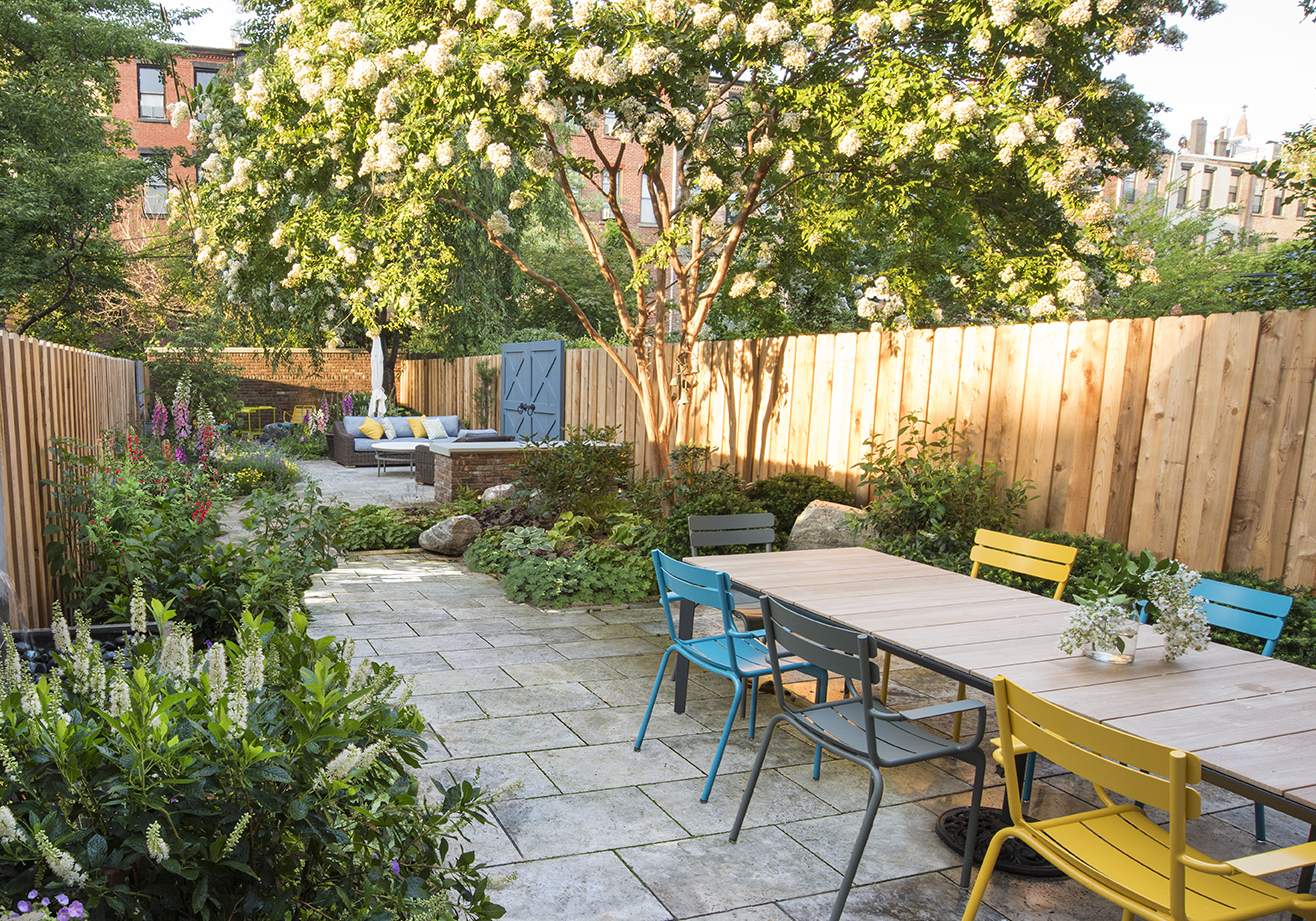The photograph captures a fenced-in outdoor patio area, likely a backyard or a side yard adjacent to an apartment complex, taken during the daytime. The yard is fairly large in depth but not particularly wide and is enclosed by a tall wooden fence made of vertical brown slats that are slightly shorter than the average human male. The floor is covered in gray rectangular concrete tiles.

Prominently featured is a long table situated on the right side of the image, surrounded by seven metal chairs in various colors including gray, blue, and yellow. Towards the back, there appears to be a cozy lounge area with a wicker couch adorned with colorful throw pillows, complemented by an additional round table.

All along the edges of the yard, a variety of bushes, shrubs, and potted plants add a lush green touch, accentuated by flowers in multiple colors such as red and purple. There's a notable large tree with white blooms, surrounded by more bushes. Toward the right, a vividly blue-painted gate offers an exit from the yard. Beyond the fence, larger buildings and additional trees are visible, indicating a residential setting, possibly surrounded by apartment complexes.